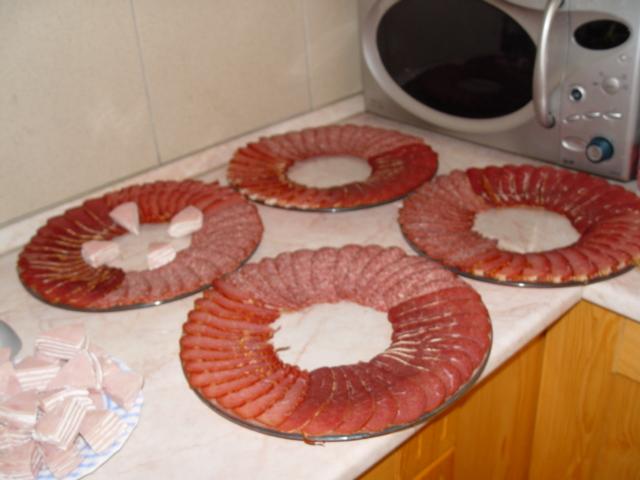The image captures a neatly arranged kitchen counter against a white tiled wall. The countertop, designed to mimic marble, is a white laminate with subtle patterns, situated in the corner of the kitchen. Oak wood cabinets with an orange-ish hue are visible underneath, while a compact microwave, silver with black accents and a prominent blue knob, sits on the far right. 

On the counter, there are four circular platters of overlapping sliced meats, including varieties like salami, pastrami, and dried beef. Each platter exhibits the same meticulous circular arrangement with a hollow center. One of these platters, distinct from the rest, has an inner display comprising four triangular stacks of what seems to be turkey meat and possibly cream cheese. 

Additionally, a plate of triangular slices, presumably cheese, is placed on the left side of the countertop, perhaps still being arranged to complement the meat platters. Together, these elements create a cohesive and visually appealing spread on the countertop.